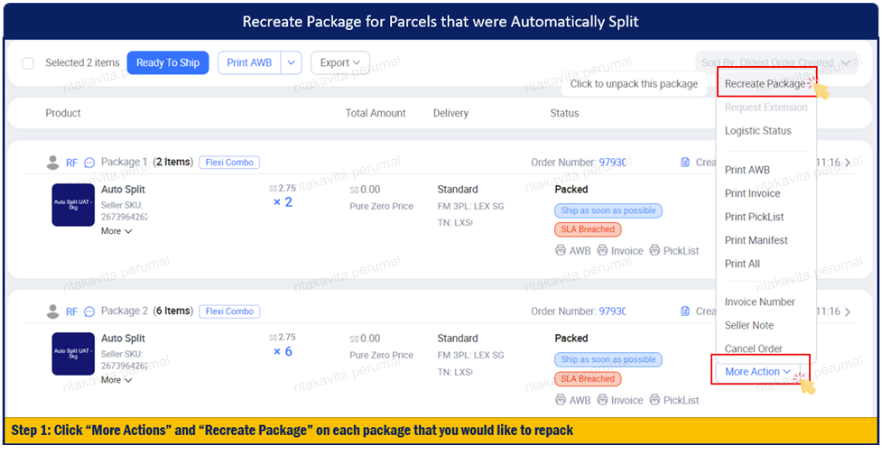The image showcases a detailed user interface for managing parcels that have been automatically split. At the top, there is a blue header with white text, indicating the different sections of the interface. Below it, checkboxes are present, showing "Selected 2 items, ready to ship" within a blue rectangle. 

Following this, there are actionable buttons such as "Print AWB" (Air Waybill) in blue text on a white rectangle, and "Export." The interface also includes detailed metrics such as "Product Total Amount" and "Delivery Status."

There is an important section highlighted by a red rectangle with a yellow arrow pointing towards it, indicating the option to "Recreate Package." Additionally, there is a pop-up bar offering a variety of print and action options— "Print AWB," "Print Invoice," "Print Pack List," "Print Pick List," "Print Manifest," and "Print All"—each available in capital letters. The interface also provides functions to manage orders, including "Invoice Number," "Seller Note," "Cancel Order," and a "More Action" option in blue, surrounded by another red rectangle with a yellow arrow.

At the very bottom, a yellow rectangle guides the user with the instruction: "Step 1: Click 'More Actions' and 'Recreate Package' on each package that you would like to repack."